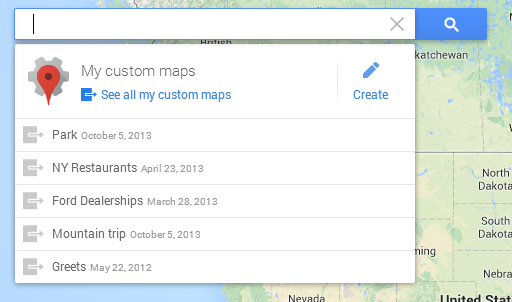**Google Maps Custom Maps Settings Interface**

The image displays a section of the Google Maps interface dedicated to managing custom maps. At the top of the interface, a search bar is prominently featured, accompanied by a blue magnifying glass icon and a close button. Just below the search bar, there's a settings icon next to a red location pin icon, immediately followed by the heading "My Custom Maps."

Beneath this heading, there is an option in blue text that reads "See all my custom maps." Adjacent to this option is a blue line labeled "Create," with the word "Create" also in blue.

The interface then lists several saved custom maps, each marked with a date:
- "Park - October 5th, 2013"
- "New York Restaurants - April 23rd, 2013"
- "Ford Dealerships - March 28th, 2013"
- "Mountain Trip - October 5th, 2013"
- "Grocery Stores - May 22nd, 2012"

This section serves as a hub for users to access, manage, and create their personalized maps, including saved locations and routes. It allows users to switch between their custom maps based on their current location or travel plans.